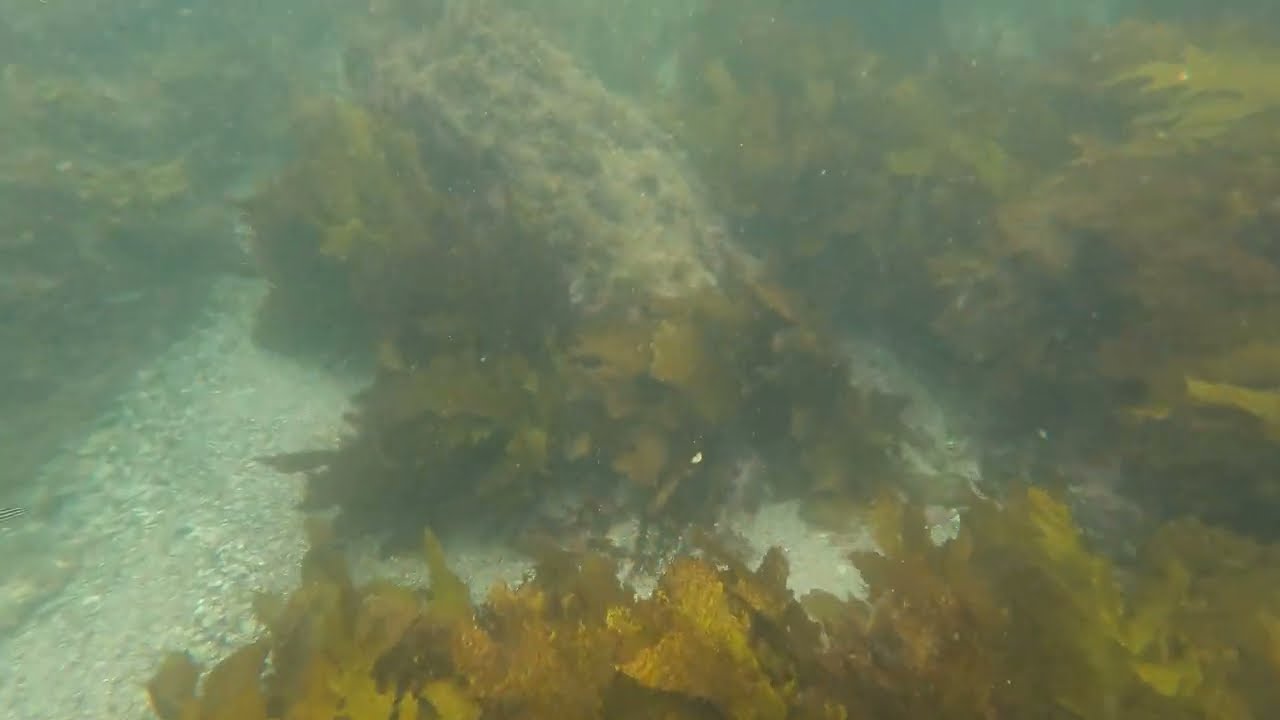An impressionistic, aerial view of an underwater seascape is depicted in this image, creating an enigmatic blend between a painting and a photograph, possibly processed to achieve an unusual perspective. The scene features murky, hazy blue water with sediment and specks, while the seafloor below is scattered with seagrass, sand, and indistinct rocks. In the foreground on the right, the thick density of seagrass and small rocky patches stands out, though everything appears somewhat blurred, lending the image an impressionistic quality. A solitary silverish fish swims near the center, contributing to the mysterious ambiance of this oceanic landscape. This combination of natural elements and artistic processing makes the scene resemble something you might find in a museum.